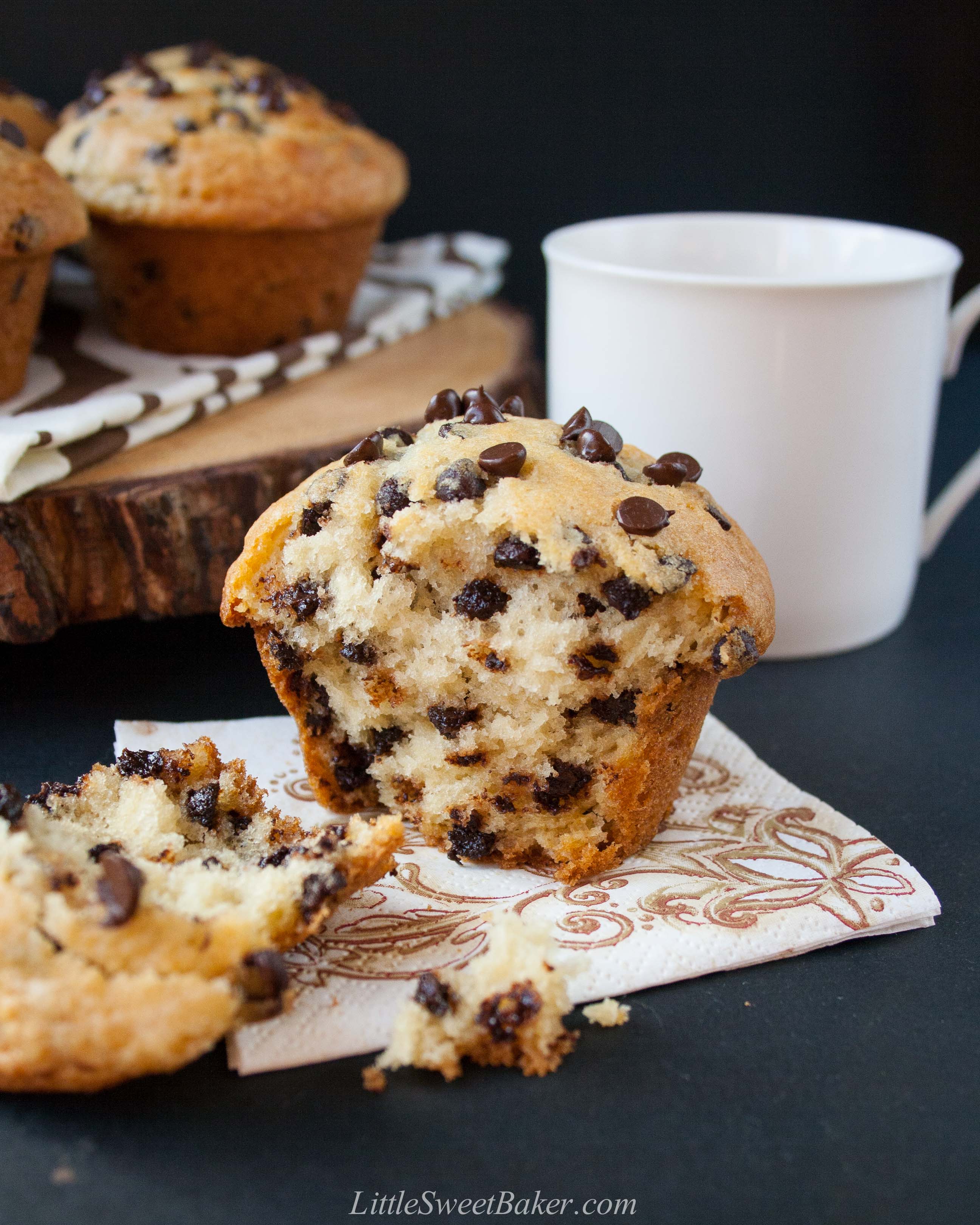The image features a delectable arrangement of miniature chocolate chip muffins. The focal point is a partially crumbled muffin on a white napkin adorned with a delicate gold filigree pattern. The torn edge reveals a lighter, beige interior contrasting its golden brown exterior speckled with abundant miniature chocolate chips. Crumbs and a large chunk of the muffin are scattered in the foreground. This setup rests on a dark, slate-colored surface, possibly a countertop or tablecloth. Behind the crumbled muffin, a pristine white coffee cup stands adjacent to a rustic wooden platter with natural bark edges. A brown and white kitchen towel is draped over the platter, which holds several intact, golden brown muffins studded with chocolate chips. The overall composition creates a cozy and inviting scene, emphasized by the rich textures and warm tones. The image is branded with a watermark at the bottom, littlesweetbaker.com.